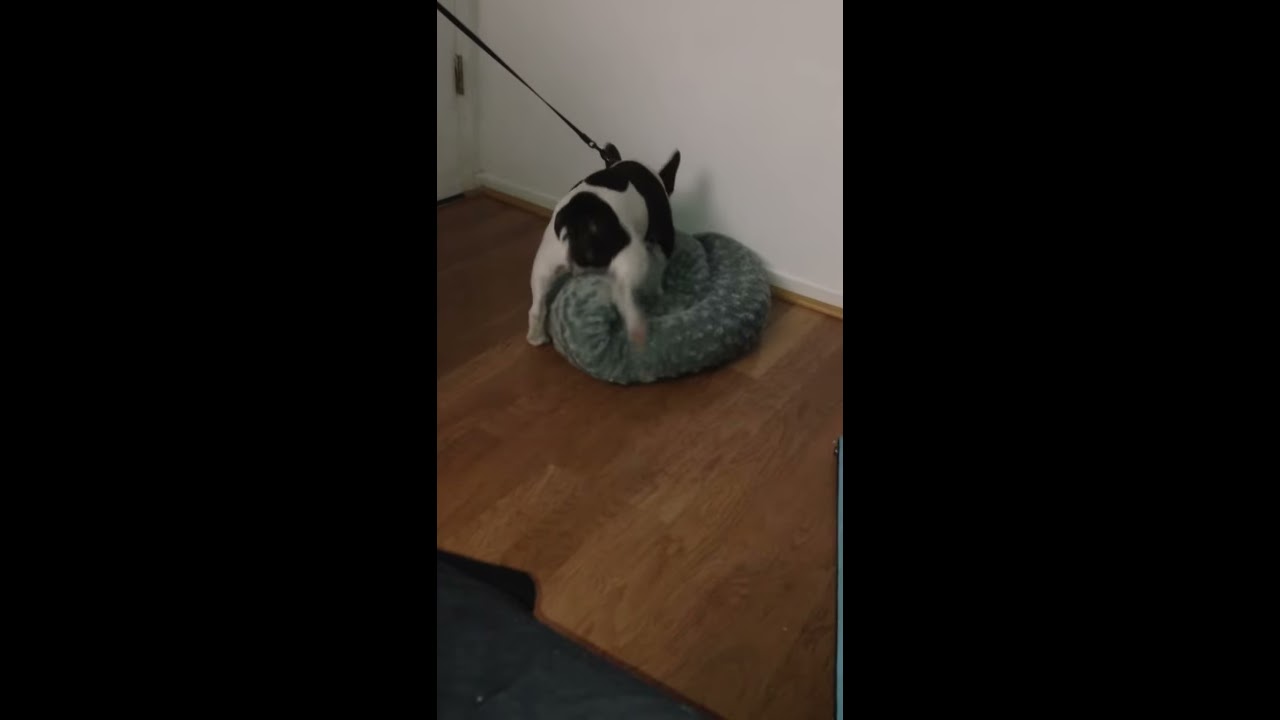This photograph, taken indoors in portrait orientation, captures the backside of a small, chubby black and white dog standing on a dark teal, well-textured doggie bed or cushion. The dog's body is mostly black with some white on its legs and a small section of its back. It has pointed, upright ears that are black. The dog is wearing a collar and attached to a black leash, which extends out of the frame, suggesting that someone out of view is holding it. The floor is made of brown wooden panels with a visible grain design, complemented by shoe molding along the base of the white wall. To the left of the image, a door with a metal latch or hinge is partially visible. In the bottom left corner of the frame, there appears to be a black mat or pad on the floor.